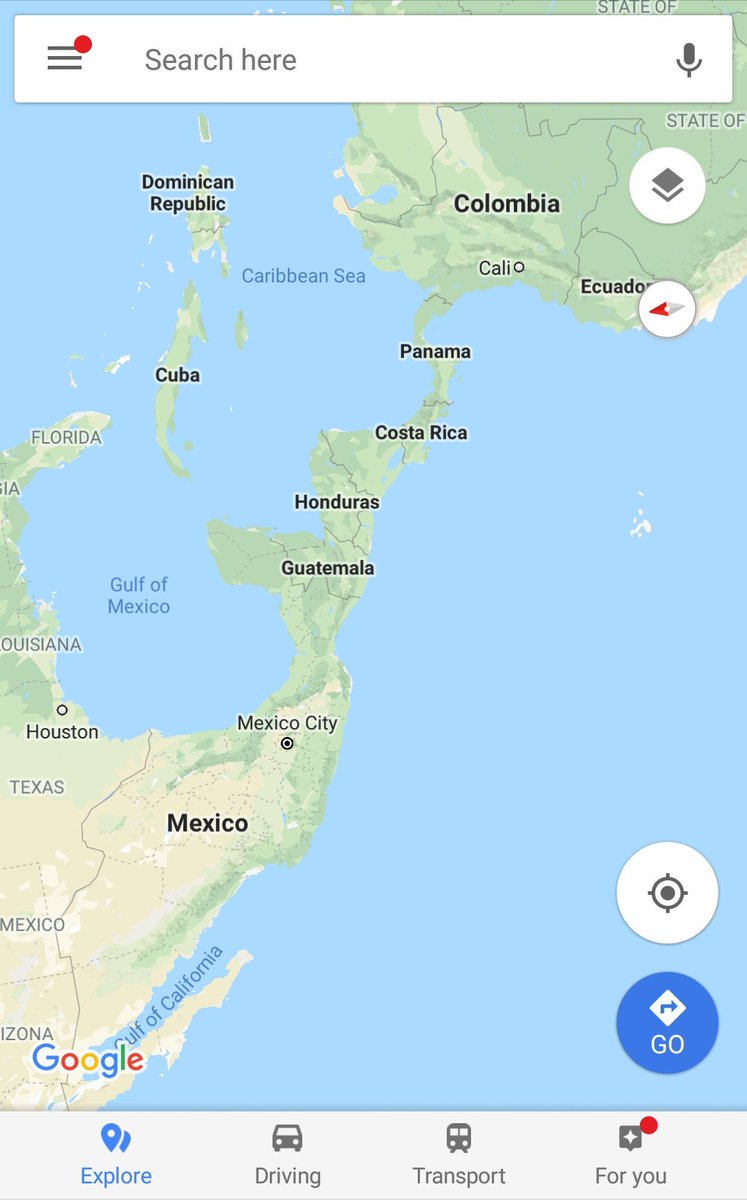This image is a screen capture from Google Maps. At the top of the image, there is a white search box featuring three gray horizontal lines, a red dot, and the prompt "Search here" in gray. The microphone icon is also gray. The map itself displays a large expanse of light blue water and green landmasses. The landmasses represent parts of Mexico, Texas, and Arizona, extending to Central America with labels for Guatemala, Honduras, Costa Rica, Panama, and the Caribbean islands including Cuba and the Dominican Republic.

The labeled bodies of water include the Gulf of Mexico, the Caribbean Sea, and the Gulf of California in gray text. At the bottom of the map, the multicolored Google logo is visible alongside various circular icons. One blue circle features white text, while a white circle includes gray text. Further, there are other circular icons distinguished by color, including a white and red one as well as a white and gray one.

The bottom portion of the image contains a gray strip with multiple icons. The word "Explore" appears in blue with a corresponding blue pin icon. Other gray icons include "Driving" denoted by a car symbol, "Transport" marked by a bus icon, and "For You," which displays a square with a star and a red dot beside it. There are no other significant details within this image.